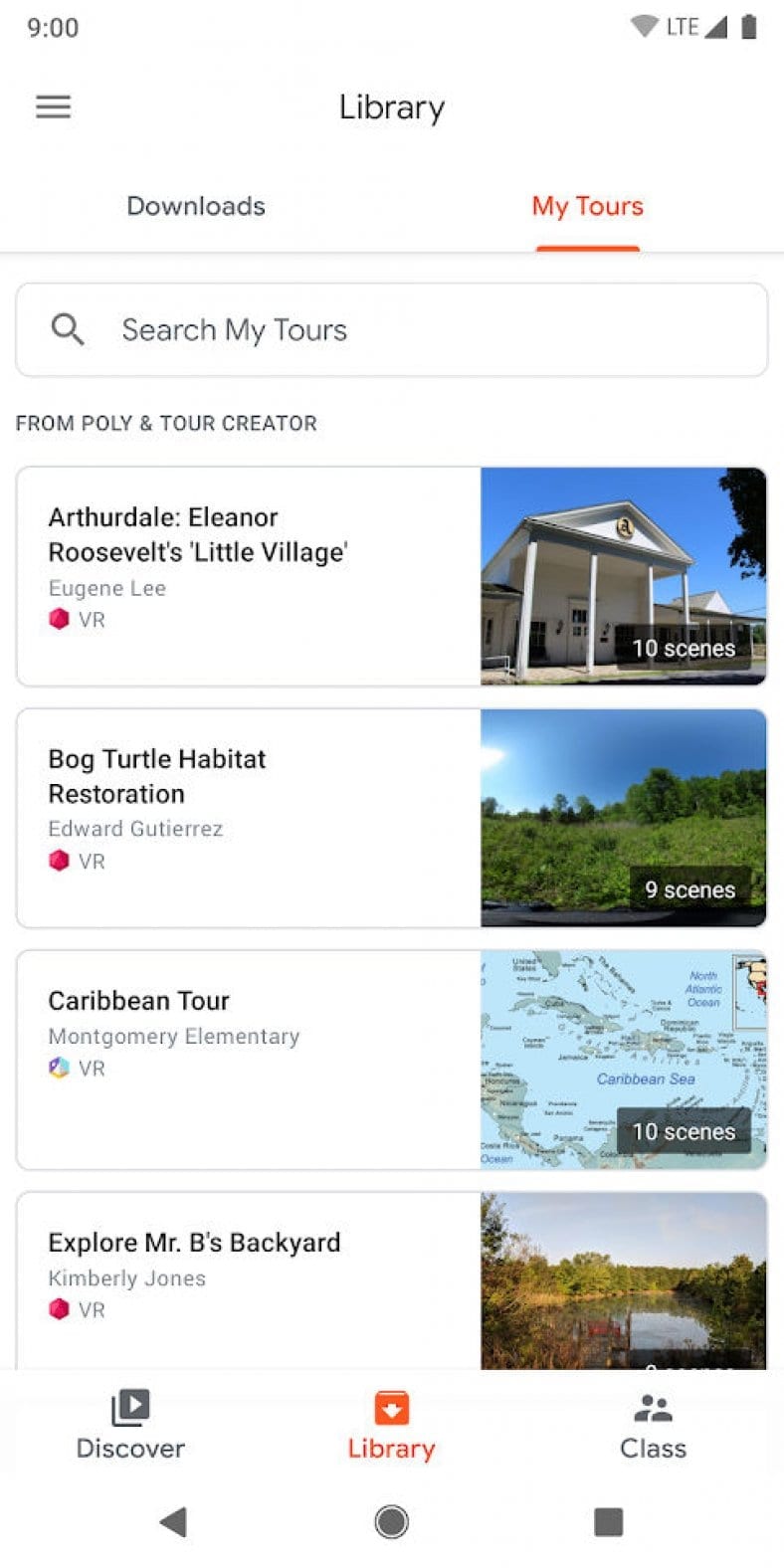A clean and detailed caption for the described photo could be:

---
This portrait-oriented screenshot captures the interface of a travel or history-themed mobile website, set against a white background, emulating the proportions typical of a cell phone screen. The status bar at the top indicates the time as 9 o'clock, full Wi-Fi and network connection, LTE signal, and a fully charged battery. Below the status bar, the header features a hamburger menu on the left and the word "Library" in the center. Under the header, two options labeled "Downloads" and "My Tours" are displayed, with "My Tours" highlighted in orange and underlined. 

A thin gray border separates the header from a long, rectangular search bar with a gray outline, labeled "Search My Tours." Beneath the search bar, the text "From Polly in Tour Creator" is displayed, followed by a list of four tours presented in long rectangular boxes. Each box has a white background with text on the left and thumbnails on the right. The tours listed are:

1. "Arthur Dale: Eleanor Roosevelt's Little Village" – a VR tour featuring 10 scenes.
2. "Bok Turtle Habitat Restoration" – also a VR tour, featuring 9 scenes.
3. "Caribbean Tour" – another VR tour, with 10 scenes.
4. "Explore Mr. B's Backyard" – a VR tour with the number of scenes not specified.

The interface’s clean design and organized layout efficiently present the various tour options available to the user.